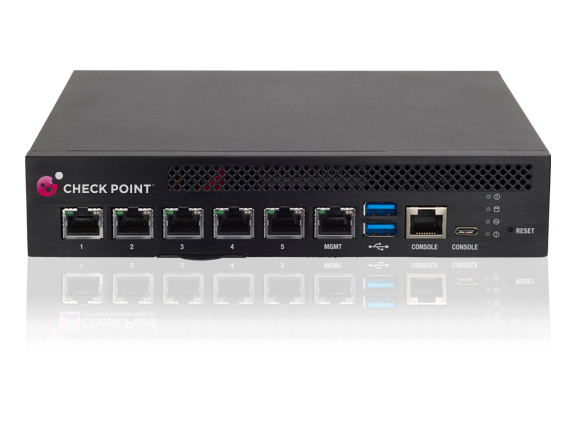The image depicts a black electronic device, likely a router or modem, positioned on a white surface. The device is notable for its sleek, black body with holes punched in the front-top section for ventilation. In the upper-left corner, a red dot and a white dot are accompanied by the word "checkpoint." The device features several input jacks: seven Ethernet ports labeled 1 through 5, with the additional labels less legible. Also present are two USB ports, a smaller USB-A or possibly USB-C port, and a port labeled "console." There is also a reset button. The overall design is typical of a product image, with a slight reflection visible on the surface beneath the device.